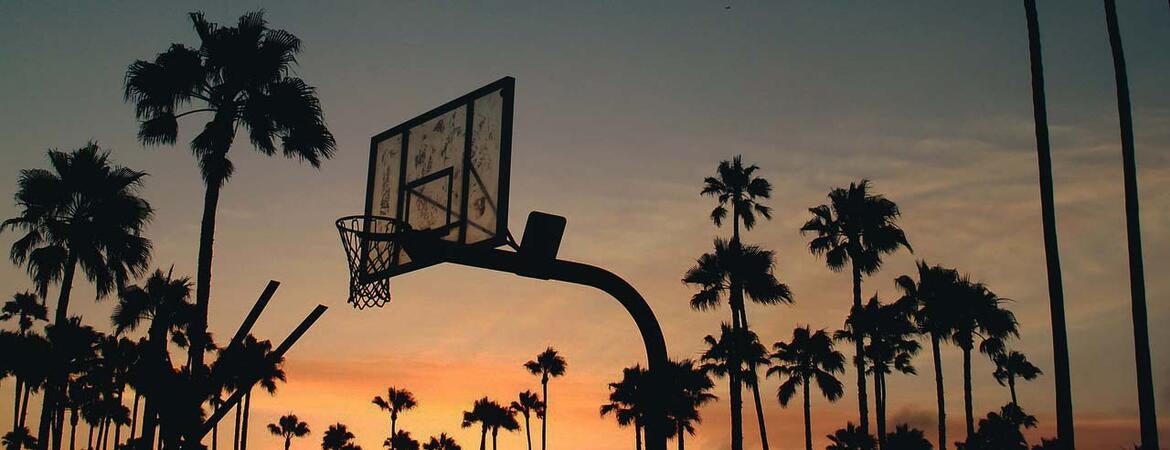The photograph captures a striking scene at dusk, featuring a central basketball hoop silhouetted against a vibrant sky. Dark blue transitions to white from scattered clouds and culminates in an orange hue from the setting sun. The sky's dramatic color gradient serves as a breathtaking backdrop. A clear plastic backboard with dark, outlined edges and center square contrasts against the sky. The metal rim holds a white net. Tall, dark palm trees, numbering around thirty and varying in height, frame the scene on either side and at the base. The trees’ silhouettes create an intriguing contrast with the colorful sky, enhancing the image’s serene yet dynamic atmosphere.